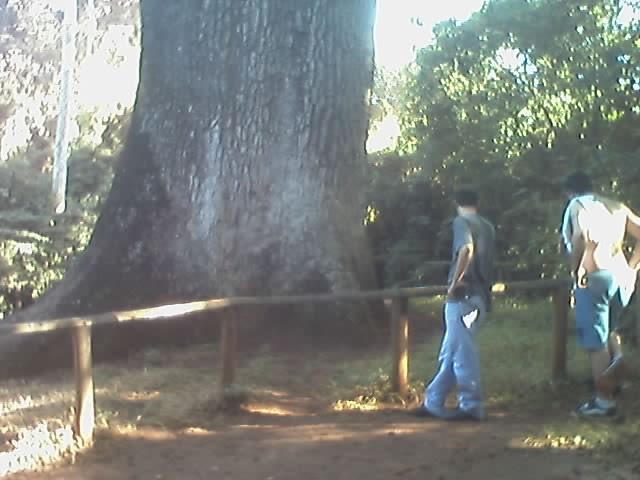Set in a park during a sunny day filtered through a light haze, this old, slightly blurry photograph, possibly from the 80s or 90s, showcases a monumental tree with a scaly trunk that spans roughly eight to ten feet in diameter. The tree, enclosed by a wooden fence with posts spaced five feet apart, stands as a notable landmark, attracting the attention of two men. One man, dressed in a white t-shirt and blue shorts with running shoes, stands next to a dark-haired man in a gray t-shirt and blue jeans. Both are positioned on a dirt path just before the fence, seemingly engrossed in observing something near the tree's base. The background is filled with other sunlit trees, some with white trunks, adding depth to the scene. The photograph's low resolution and old-fashioned appearance suggest it was captured with an outdated camcorder, adding to its nostalgic charm.